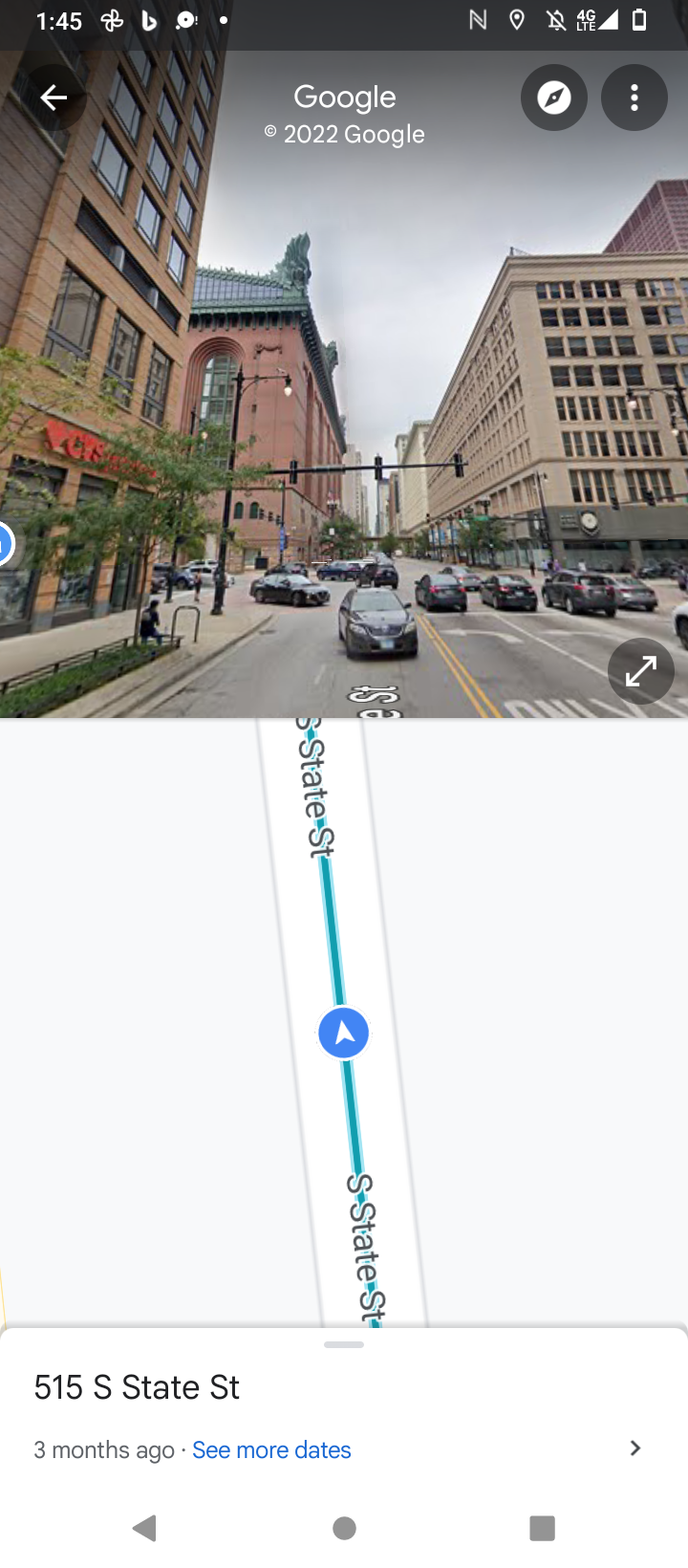The image depicts a smartphone screen showing a detailed 3D map. The top half of the screen displays the live view of the map with notification icons populating the status bar on the right side. These icons include a white padlock, full bars of 4G signal, a diagonal line symbolizing silence mode, a white location icon, and several other icons.

On the left side of the status bar, the time is shown as 1:45, alongside fan and ping logos, a storage full icon, and a dock icon, all in white. At the center of the map is the text "gookly copyright 2002 gookly" in white.

The road on the map has two lanes with various cars approaching the center of the image from different directions, including some from the east. There are houses situated on both sides of the road; the house on the right is light brown, while the one on the left is maroon. Another brown house is located on the bottom left, and there is a red log positioned among trees in the foreground.

On the bottom part of the screen, the map provides directions with a blue circle and a white arrow indicating the route, leading upwards towards the top. The location is marked as "512 State St three months ago." Below this, there's a "See more" label and a gray arrow pointing left. In the center bottom, there is a gray circle, and on the bottom right, there is a gray square.